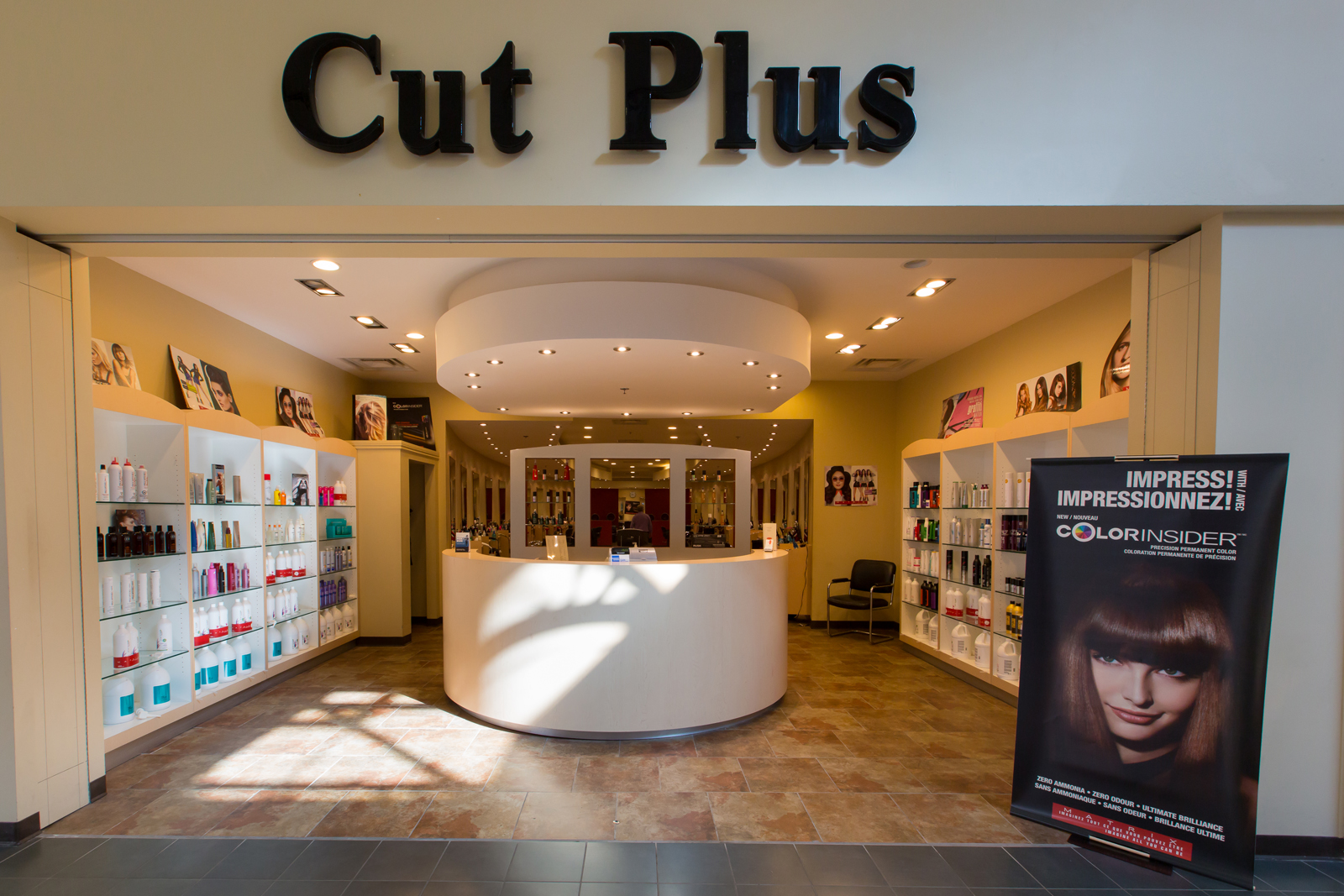The image depicts a hair salon named "Cut Plus" located inside a mall, prominently identified by its large black-lettered sign above the entrance. Outside the salon, there is a notable advertisement featuring a woman with brown, bob-styled hair, set against a black background with white writing that reads "Color Insider." The exterior also features black tiles and a beige facade, along with a gray-tiled border marking the walkway area.

Inside the salon, beige and tan marble flooring complements the overhead lighting that illuminates a circular white reception desk equipped with a computer screen. The left and right walls are lined with white shelves displaying a variety of hair products in bottles of different colors, including white with red and blue, as well as black and yellow. Above these shelves, photographs showcase women with various hair colors and styles. Additionally, a chair is positioned in the right corner near the reception area. The back section of the salon, though not clearly visible, is presumed to be the area where hair styling takes place.